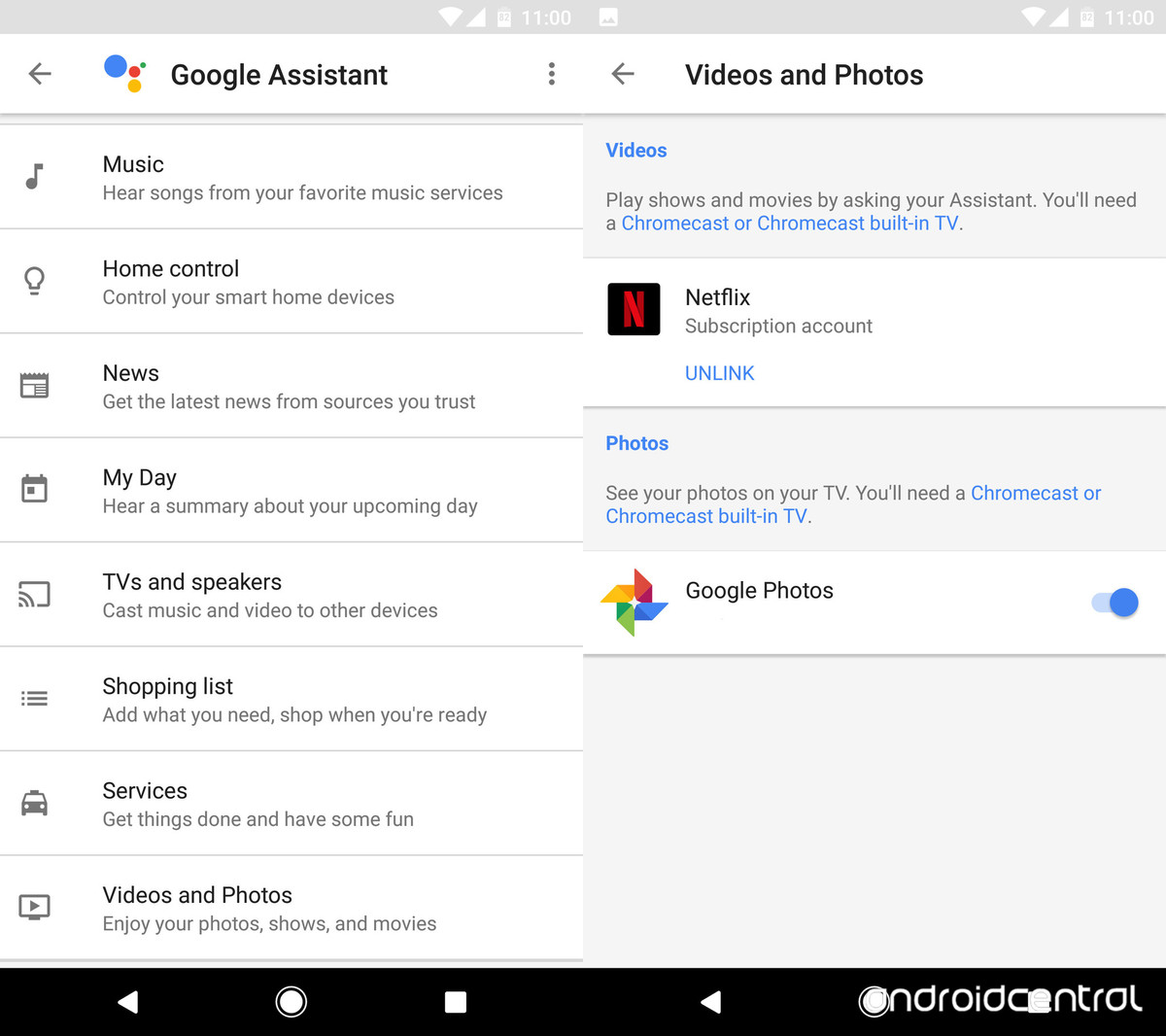This is a detailed screenshot of the Google Assistant menu interface. At the very top of the screen, there is a gray status bar displaying various system information including white icons for Wi-Fi, mobile signal strength, and a battery icon showing 82% charge. The time is displayed as 11:00. To the right of these icons, there is an additional icon for photo notifications.

Directly below the status bar, there's a white header banner. On the left side of this banner, 'Google Assistant' is written in black font, and next to it is the Google Assistant logo consisting of four multi-colored circles. An arrow pointing to the left appears next to the logo, indicating a navigation option. Toward the right side of this banner, there are three vertical dots that signify additional menu options, followed by another left-pointing arrow. Further to the right, 'Videos and Photos' is displayed in black font, suggesting a subsection of the Google Assistant menu.

Beneath this header, the primary content of the menu is displayed. The menu consists of eight vertically aligned options, each within a white rectangular button. At the top of the list, 'Music' is written in black font, followed by the description 'Hear songs from your favorite music services'. The next option is 'Home Control', accompanied by the description 'Control your smart home devices'.

The detailed visual and textual elements of the interface provide a clear layout and functionalities available within this specific section of the Google Assistant menu.